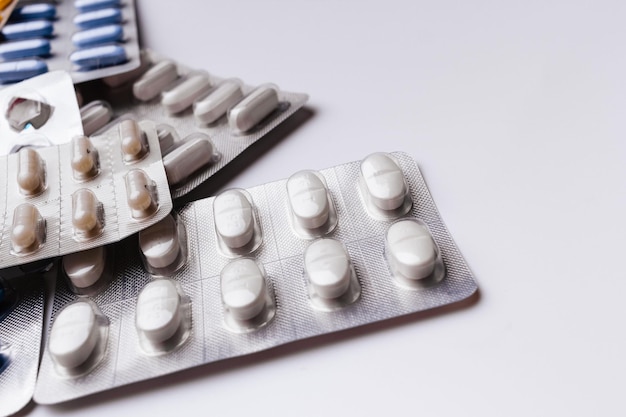The photograph depicts an assortment of medicinal products still encased in their foil wrappers. The background is a light gray, providing a neutral backdrop that highlights the various colors and forms of the pills. Central to the image, the packages are stacked on top of each other, with the sequence running from right to left. Dominantly featured at the top left are oval-shaped blue capsules, which are followed by a mixture of other pills in descending order.

In total, there are several blister packs visible. The forefront features a tab containing ten round white tablets. Above it, another tab displays six visible capsules. Further up, another tab of capsules is evident, continuing the layered arrangement of medicinal products. The pills vary in form and color, ranging from white to tan, blue, and red capsules. Among them, capsules and solid tablet forms are distinguishable, each designed for specific medicinal purposes. The image's arrangement showcases the chaotic yet organized nature of medicinal storage, emphasizing the diversity in pharmaceutical products.